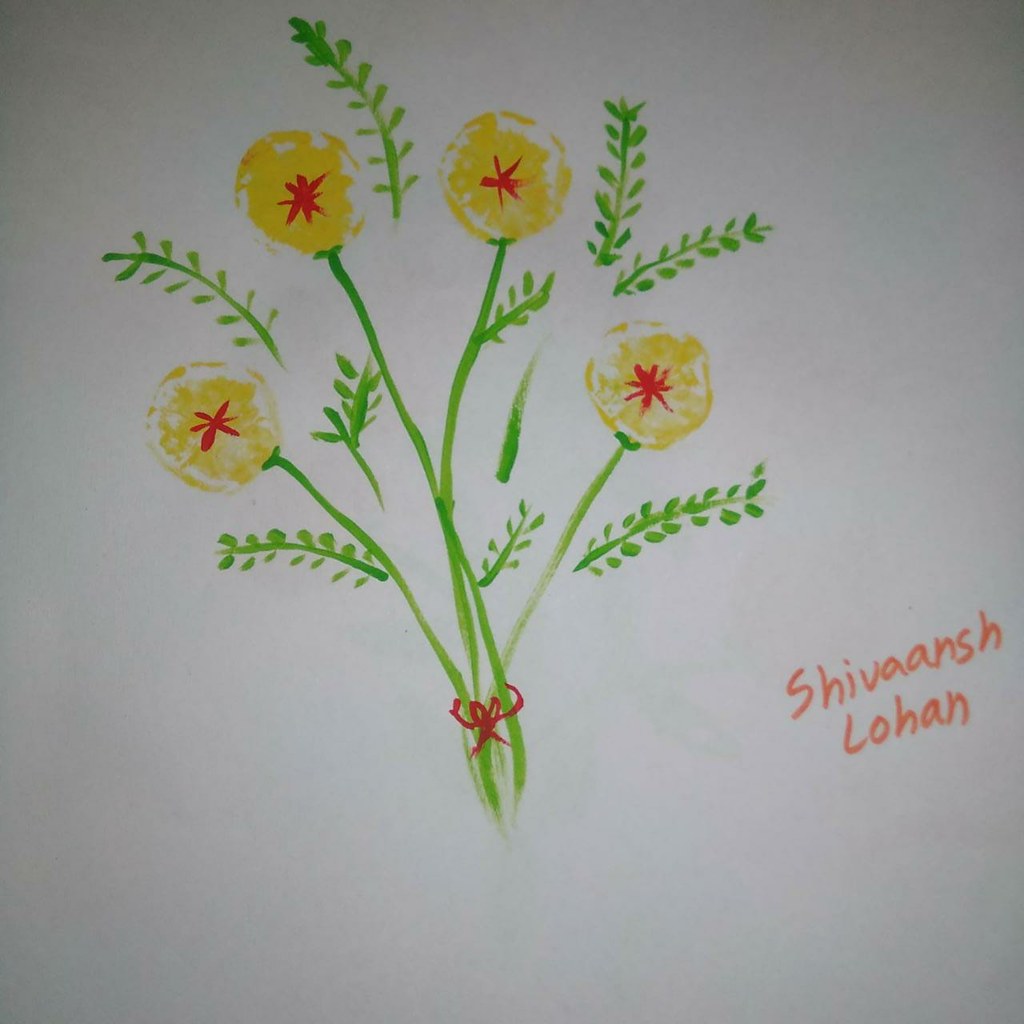This image depicts a detailed sketch on a very large white piece of paper, likely rendered with felt tip pens. The focal point is a bouquet composed of long green stems with numerous leaves resembling those of ferns, characterized by a central stem with many tiny leaves on either side. The flowers, prominently yellow with a glossy appearance, are concentrated around the sides and feature a distinctive red star at the center. There are four such yellow flowers extending from the upper branches. The bouquet is neatly tied together with a red ribbon, securing the stems at the bottom. The child's name, "Sivansh Lohan," is written in orange to the right side of the bouquet. The top two edges of the paper are shaded dark, adding a subtle frame to the illustration.